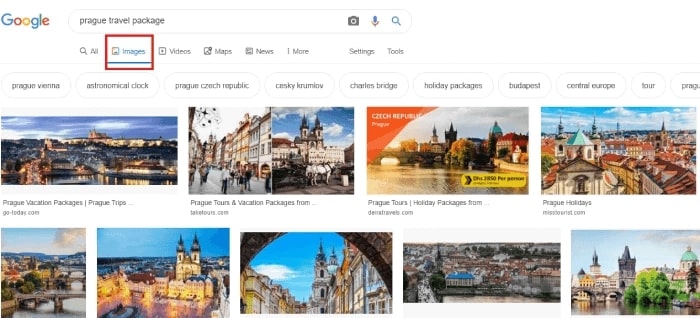A detailed and cleaned-up caption for the described image could be:

---

The image showcases a Google Images search result page with a crisp white background. At the top center, the Google logo is prominently displayed in its iconic colors: blue for the 'G', red for the first 'o', yellow for the second 'o', blue for the 'g', green for the 'l', and red for the 'e'. To the right of the logo, the familiar search bar is visible, featuring a camera icon for image search, a microphone for voice search, and the magnifying glass icon for initiating the search. The search query entered is "Prague Travel Package". 

Below the search bar, the navigation options "All", "Images", "Videos", "Maps", "News", and "More" are displayed, with "Images" highlighted in a red square. Underneath, suggested related searches such as "Prague", "Vienna", "Prague Czech", "Kremlin", "Charles Bridge", "Packages", "Budgets", and "Central" are listed.

The main content area displays a grid of nine vibrant images, each showcasing the breathtaking architecture and historic landmarks of Prague. The images feature stunning views of old buildings, majestic castles, and scenic tours, capturing the essence and beauty of Prague’s architectural heritage.

---

This caption provides a clear and comprehensive description of the Google search result page, highlighting the main elements and visually describing the images of Prague.